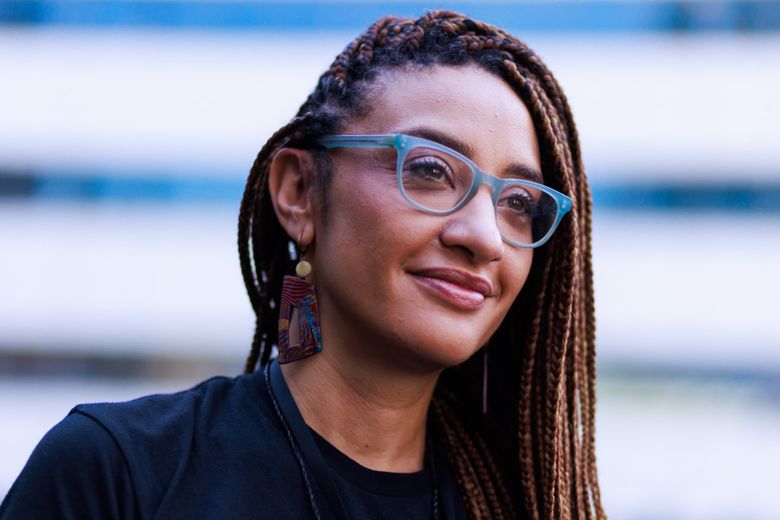This close-up image features a smiling Black woman with long, micro-braided hair, predominantly swept over to her left side, with two braids extending down her back. She wears distinctive, iridescent light blue glasses that have a slightly transparent quality. Her eyes, accented with eyeshadow and mascara, show prominently through the blue-framed glasses. Her right ear, unobscured by her hair, displays a large, dangly earring, appearing to be made of wood, featuring various colors including burgundy, blue, red, white, and black. Her attire consists of a dark, possibly navy blue t-shirt, and she has on subtle makeup, including faint lipstick. The background is light-colored and blurred, showing alternating blue and white bands that give the impression of a fence behind her.